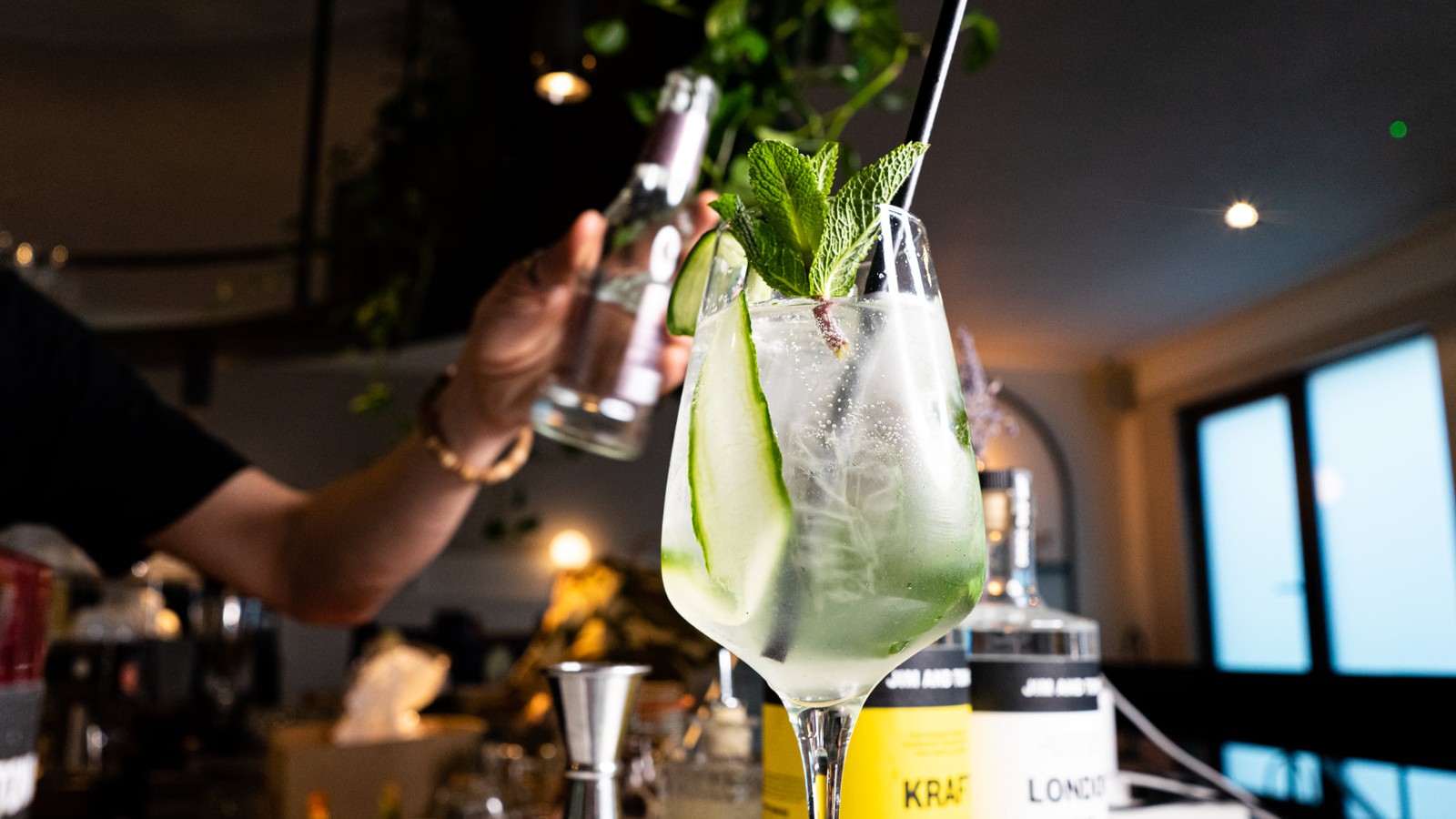In this detailed photographic image, the focus is on a refreshing cocktail prominently placed front and center. The cocktail, which could be a mojito or a cucumber mojito, is presented in a large, frosted wine glass brimming with ice and a clear, transparent liquid. Garnished with a slice of cucumber and sprigs of mint, a black straw protrudes invitingly from the glass. A person dressed in a black shirt, visible from the left side, pours a liquid from a glass bottle into the cocktail. In the sophisticated and elegant backdrop of the scene, a classy restaurant or bar setting unfolds. The right side of the frame reveals a seating area and large windows that let in soft light, while to the left, a bartender can be seen holding a bottle of liquor with a jigger resting on the bar surface. In the distance, a table with people is faintly visible, contributing to the lively yet refined atmosphere.